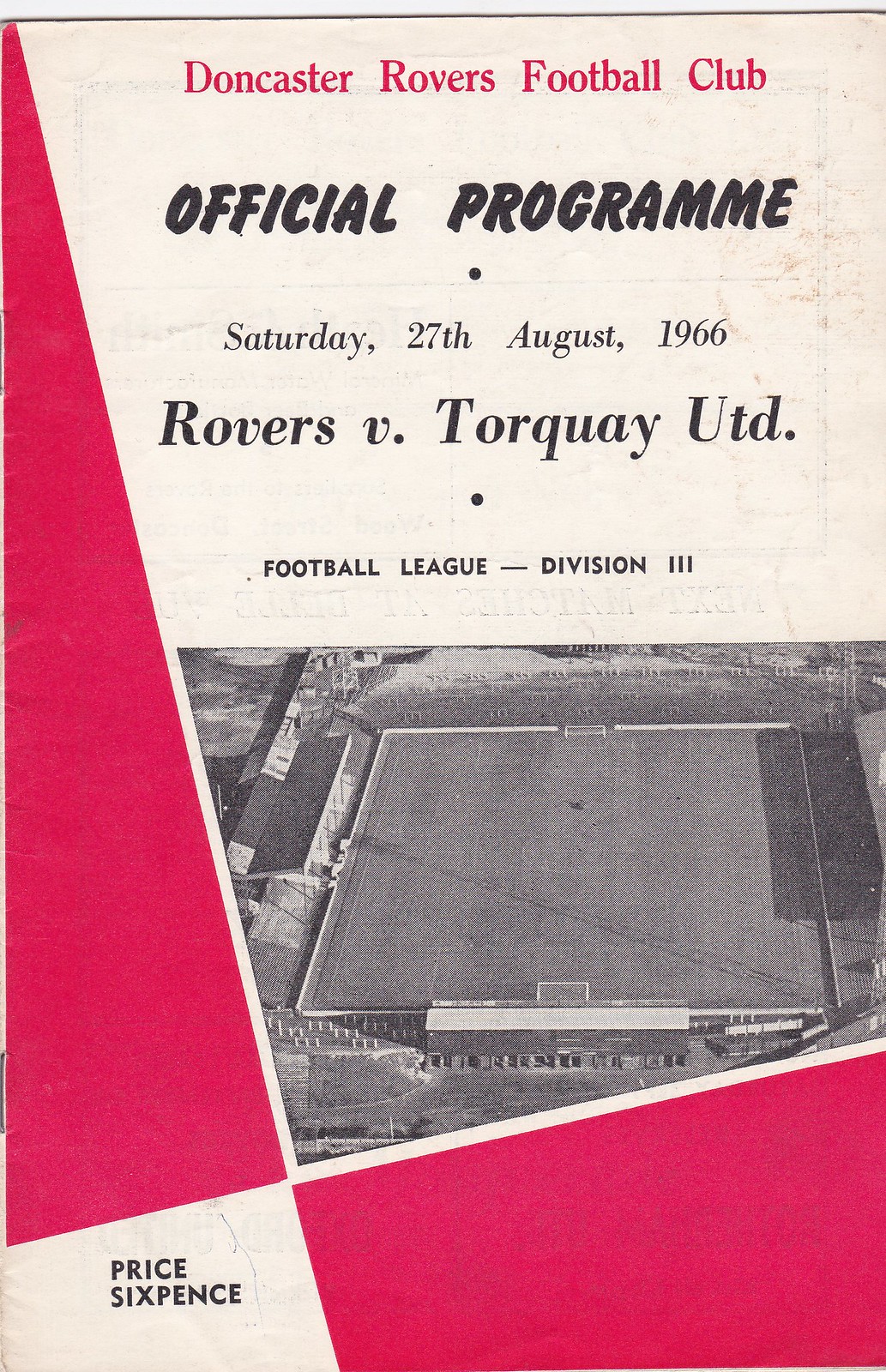The image is of an old, well-preserved football programme for the Doncaster Rovers Football Club, dated Saturday, 27th August 1966, for a match against Torquay United in Football League Division III. The programme, primarily white with signs of wear and slight dirt marks at the upper right corner, features red geometric shapes, including a triangular block to the left and an oddly shaped block in the bottom corner. At the top, in prominent red text, it reads "Doncaster Rovers Football Club," and directly beneath, in black capital letters, it states "Official Programme." Further details, such as the date and opponent, are also printed, followed by a black and white photograph of an empty, open football pitch at the center. The price of the programme, noted in the bottom left-hand corner, is six pence.